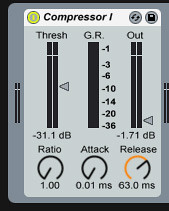The image depicts a detailed control panel for a compressor, set against a predominantly gray background with a dark black border and a darker gray inner border. The main surface, where all the information is displayed, is a lighter gray. At the top of the panel, there is a white horizontal band that prominently labels the device as "Compressor 1" in black letters, accompanied by a small logo on the left and two additional circles on the upper right side.

Below this band, there are three vertical black lines on a gray background. The left line is labeled "thresh," the middle line "G.R." with numerical markers (ranging from -1 to -36), and the right line "out." The "thresh" line reads -31.1 dB, while the "out" line registers -1.71 dB. 

Directly beneath these lines, three gauges provide further compressor measurements. These circular gauges are labeled "ratio," "attack," and "release." The "ratio" gauge has a reading of 1, and the "attack" gauge shows 0.01 ms. The "release" gauge, which is partially yellow and otherwise black, indicates 63.0 ms. Each circle contains a dial pointed at a specific level, facilitating precise control adjustments.